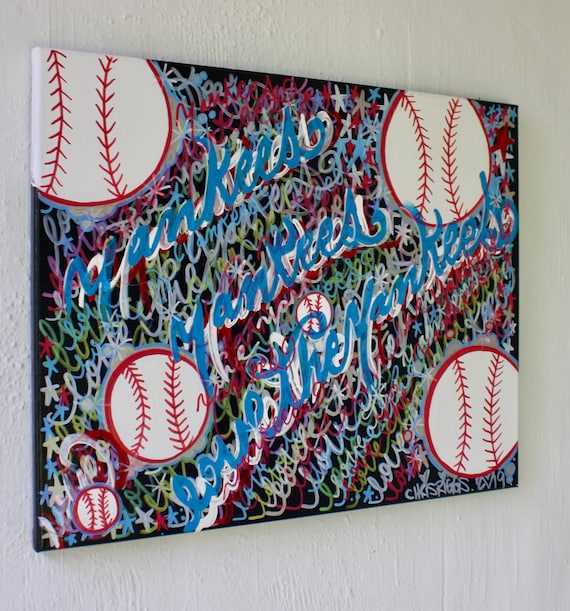The painting, dedicated to the Yankees, is displayed against an off-white wall. It features a black canvas filled with an intricate mix of text and drawings. Predominantly, in large blue cursive letters with a white shadow, it reads, "Yankees, Yankees, love the Yankees." Surrounding this central text are multiple repetitions of "love the Yankees" scrawled in red, green, and brown hues, creating a densely layered visual effect.

The artwork includes six baseballs, differentiated by size—four larger and two smaller. These baseballs are white with red stitching, meticulously detailed to resemble real-life counterparts. Multi-colored stars in red, white, and blue are scattered throughout the painting, adding a festive element.

In the lower right corner, there's a signature that appears to read "Chris Riggs," though the exact name is somewhat unclear, possibly noted as CHKS2. This signature is accompanied by the date "2019," indicating the year of creation. Overall, the bold use of color and text against the dark background makes this painting a vibrant homage to the Yankees.